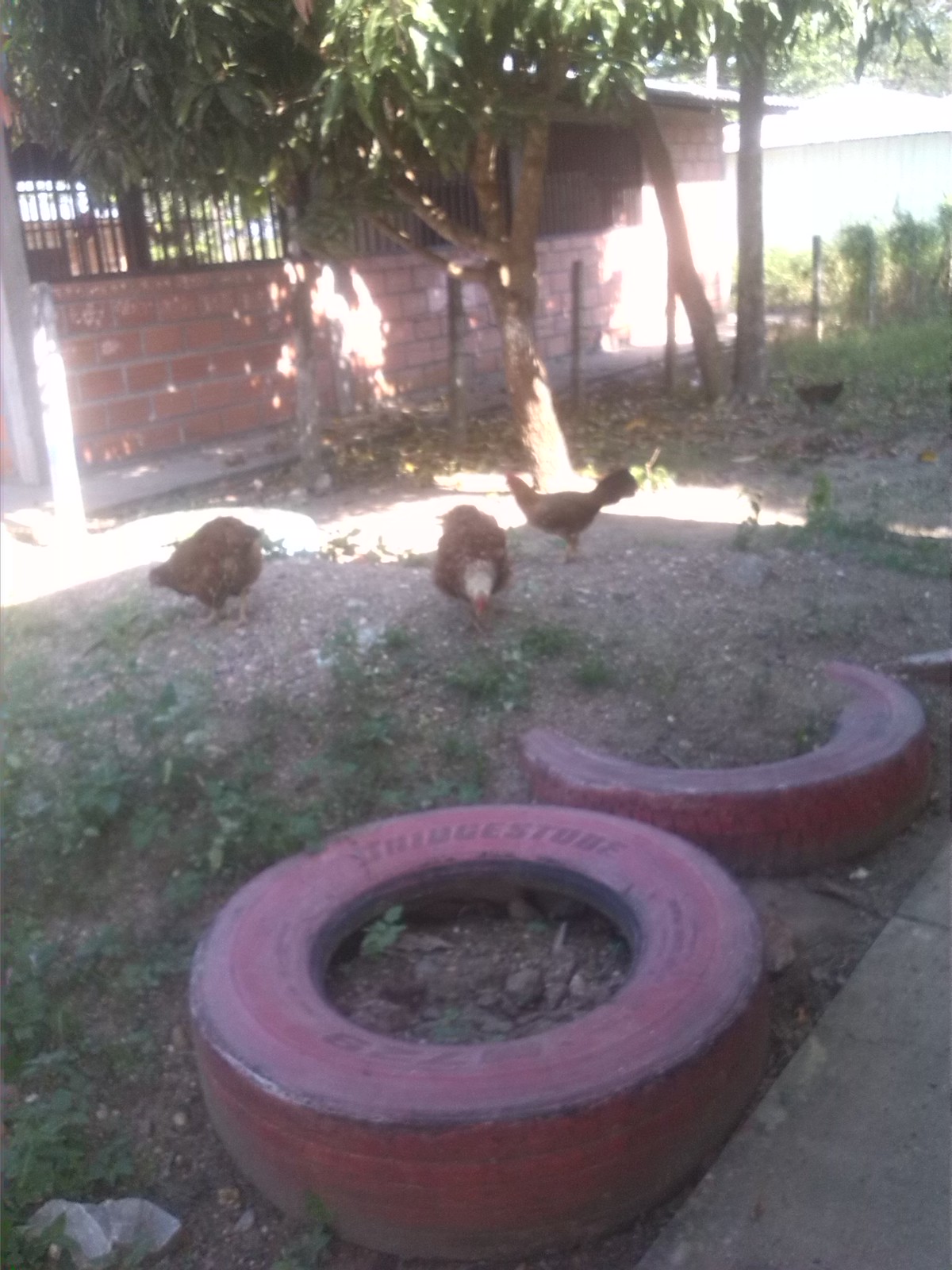This image captures a backyard scene featuring four chickens actively pecking at the ground amid a predominantly dirt and gravel terrain dotted with patches of green weeds. Positioned in the center-left, three chickens are closely grouped together, engrossed in their search for food, while a darker chicken is seen in the grassy background, also pecking at the ground. Flanking the scene are areas of greenery, including two trees with bushy green leaves, one leaning towards another building. Red-painted car tires, marked with the name Bridgestone, are partially buried in the soil near some scattered rocks, adding a rustic element to the yard. A terracotta brick wall lines the top left of the scene, with small posts visible just beyond it. In the bottom right corner, gray-tan patio paving tiles and a gray rock complete the setting, all under a canopy of shaded sunlight filtering through a thin beam, illuminating the base of a small tree. The backyard is enclosed by black gates and features additional structural elements like bushes and fences, enriching the bucolic atmosphere.